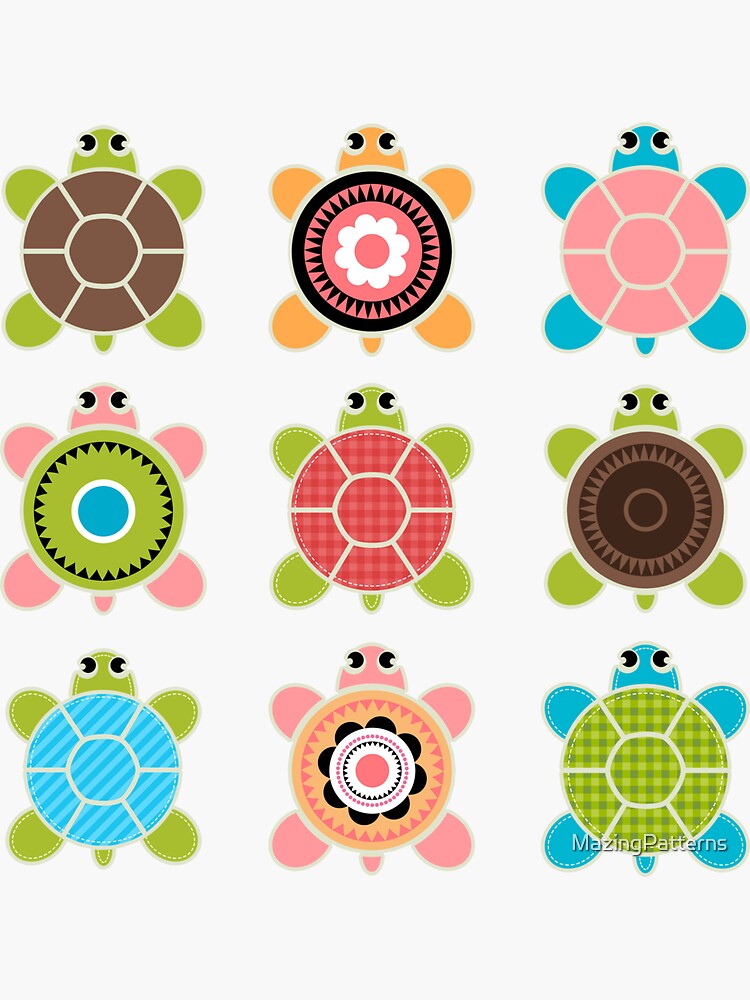This illustration features nine whimsical, cartoonish turtles organized in three rows against a white background. Viewed from above, each turtle is uniquely colorful with non-realistic hues such as pink, blue, orange, and green. The turtles' shells, perfectly round, exhibit an array of intricate patterns including flowers, stripes, gingham, and geometric shapes reminiscent of hex signs. Each shell's design contrasts strikingly with the turtle's body color, for instance, a green turtle with a brown shell or a blue turtle with a pink shell. The turtles are uniformly oriented with their heads pointing upward, and their designs include elements like circles, lines, and contrasting color schemes. At the bottom right corner, the text “Amazing Patterns” is displayed, stylized as "M-A-Z-I-N-G Patterns."